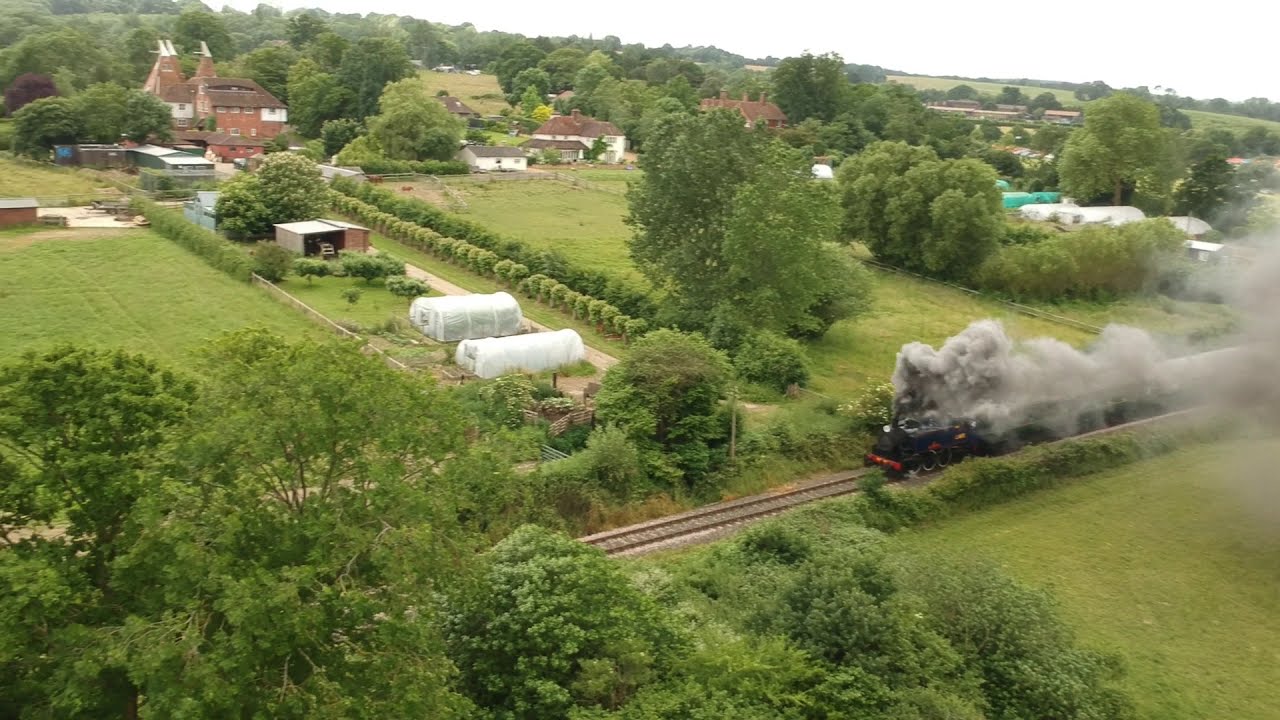This image presents a serene aerial view of a picturesque countryside dominated by vibrant green fields and grasslands. The centerpiece is a black locomotive chugging along brown railroad tracks, emitting thick gray smoke that partly obscures the train, leaving only its front visible. The scene is framed by an array of verdant trees and shrubs, with some green crops covered with white tarps or film adding contrast to the landscape.

In the upper left corner and background, you can spot a few houses and potential grain storage structures, suggesting a blend of residential and agricultural use. Notably, there's a larger shed-like building with a white roof and several brick houses with brown roofs, accompanied by cars parked in driveways. Additional structures with bluish or greenish and white appearances are visible on the right side, though their exact purpose remains unclear.

The tranquil landscape is peppered with trees and bushes that circle the entire image, and the sky above is a muted white, enhancing the tranquil and idyllic vibe of this countryside scene. It's a beautiful blend of natural and human-made elements that evoke a sense of peaceful rural life.